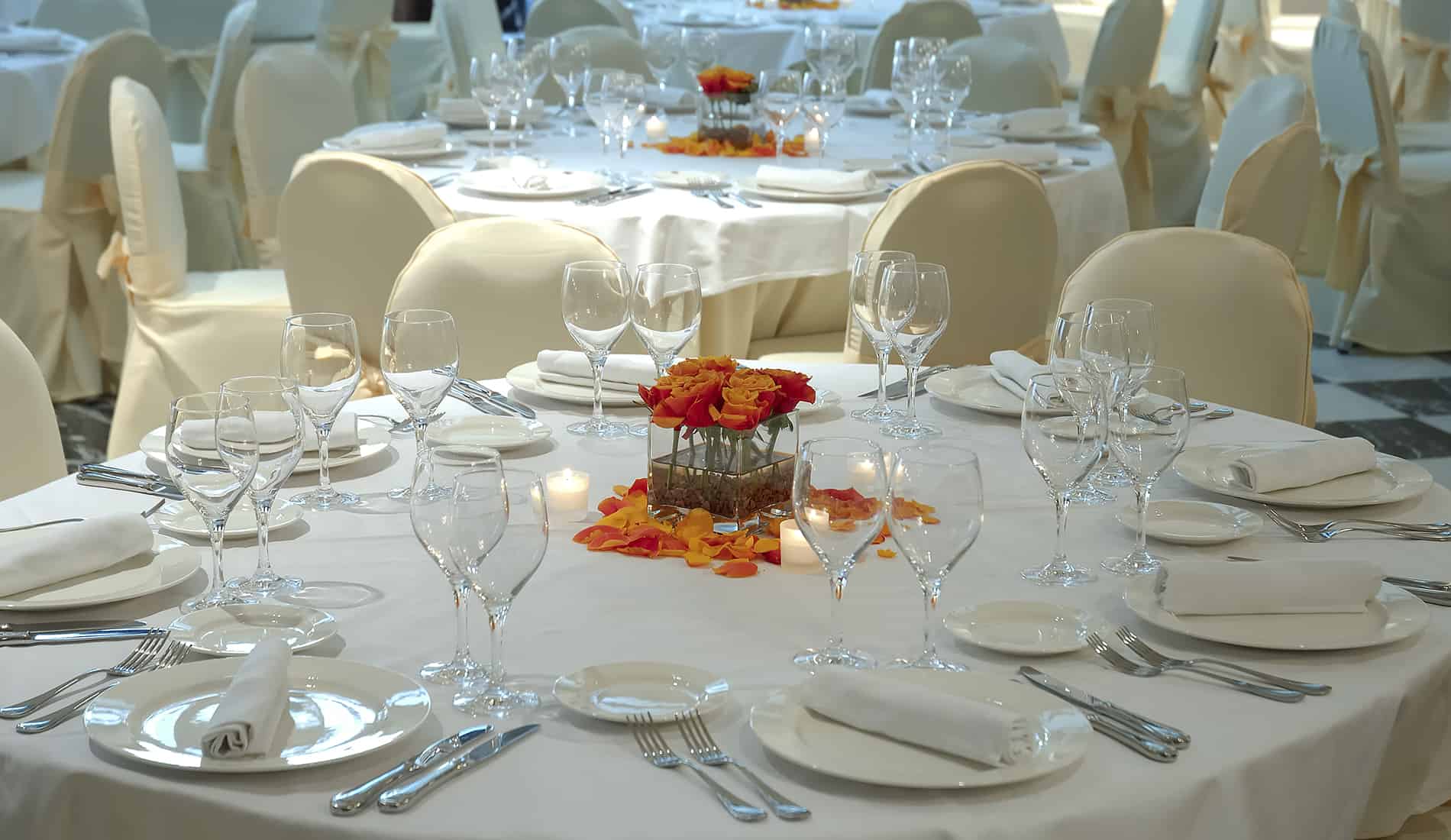This photograph captures the elegant setup of a fancy dinner event inside a Union venue, possibly prepared for a wedding reception. The image is centered around round tables, each adorned with pristine white tablecloths and meticulously arranged place settings. A prominent table in the forefront showcases settings that include white plates and small saucers, with neatly folded white napkins placed in the center of each plate. Each place setting features two forks positioned on the left and two knives on the right, accompanied by two wine glasses in front.

The chairs around the tables are elegantly wrapped in a white cream material, giving the appearance of neatly tied presents. The tables' centerpieces are beautifully arranged with red and orange roses, accented by scattered rose petals. The scene is complemented by multiple candles that enhance the romantic ambiance.

In the background, additional tables are visible, maintaining the same sophisticated decor, suggesting a lavish and carefully planned event designed for a large number of guests. The overall aesthetic is one of refined elegance, with attention to detail evident in every aspect of the table settings and decorations.